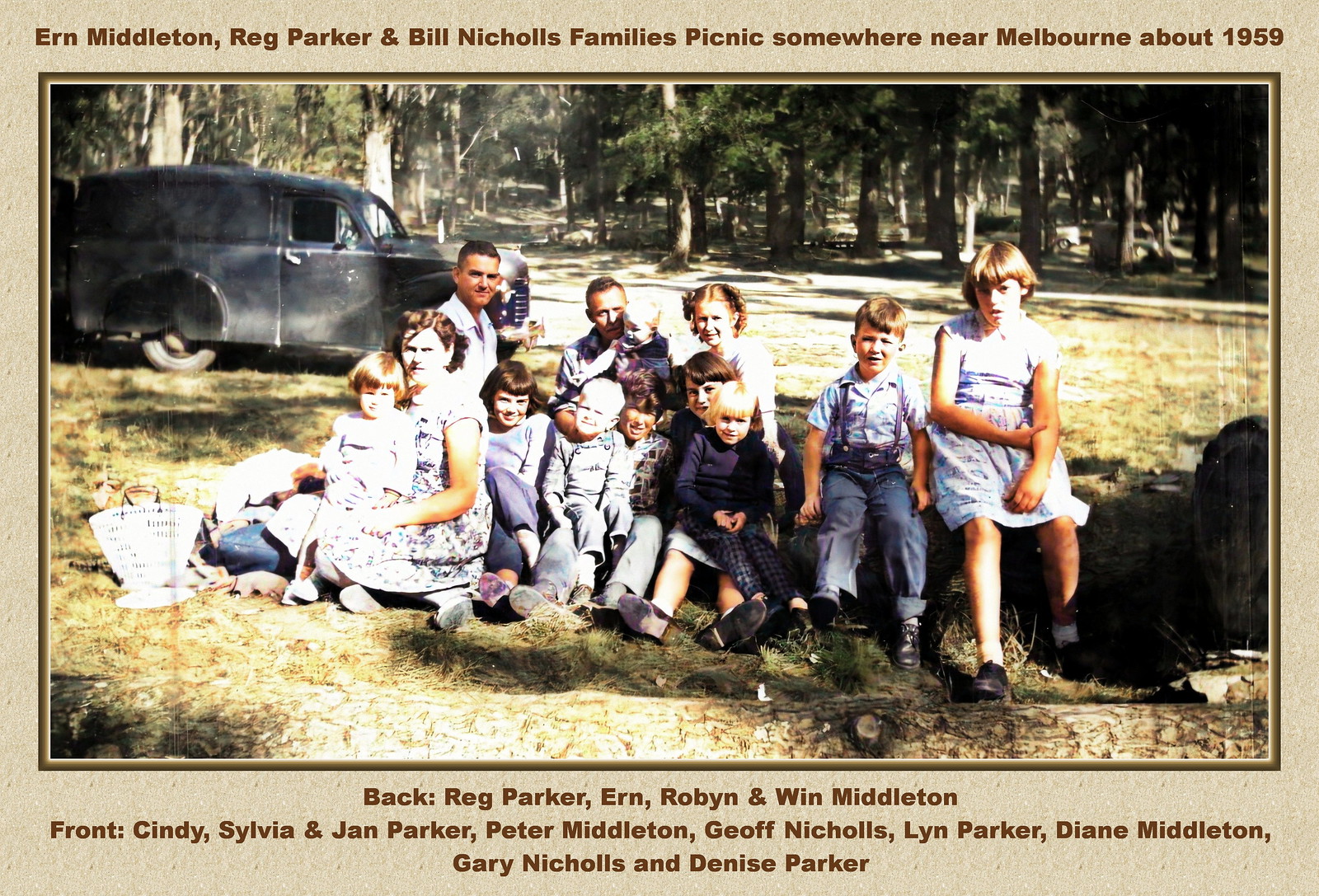The rectangular photograph captures a large family gathering at what appears to be a woodland picnic area or campground near Melbourne, around 1959. The setting is rustic, with a long log on the ground that some family members are sitting on. Behind the group, an old-fashioned black car or truck serves as a backdrop, further emphasizing the time period. The detailed attire suggests the era, with boys in suspenders, rolled-up jeans, and black boots, while the girls wear dated dresses. The top of the photograph bears the inscription: "Erne Middleton, Reg Parker, and Bill Nichols' family's picnic somewhere near Melbourne, about 1959." The bottom lists the individuals: "Back: Reg Parker, Erne, Robin, and Wynne Middleton. Front: Cindy, Sylvia, and Jan Parker; Petal Middleton; Jeff Nichols; Lynn Parker; Diane Middleton; Gary Nichols; and Denise Parker." The combined families, potentially as many as a dozen children, embody the close-knit, multi-generational family outings of the 1950s.